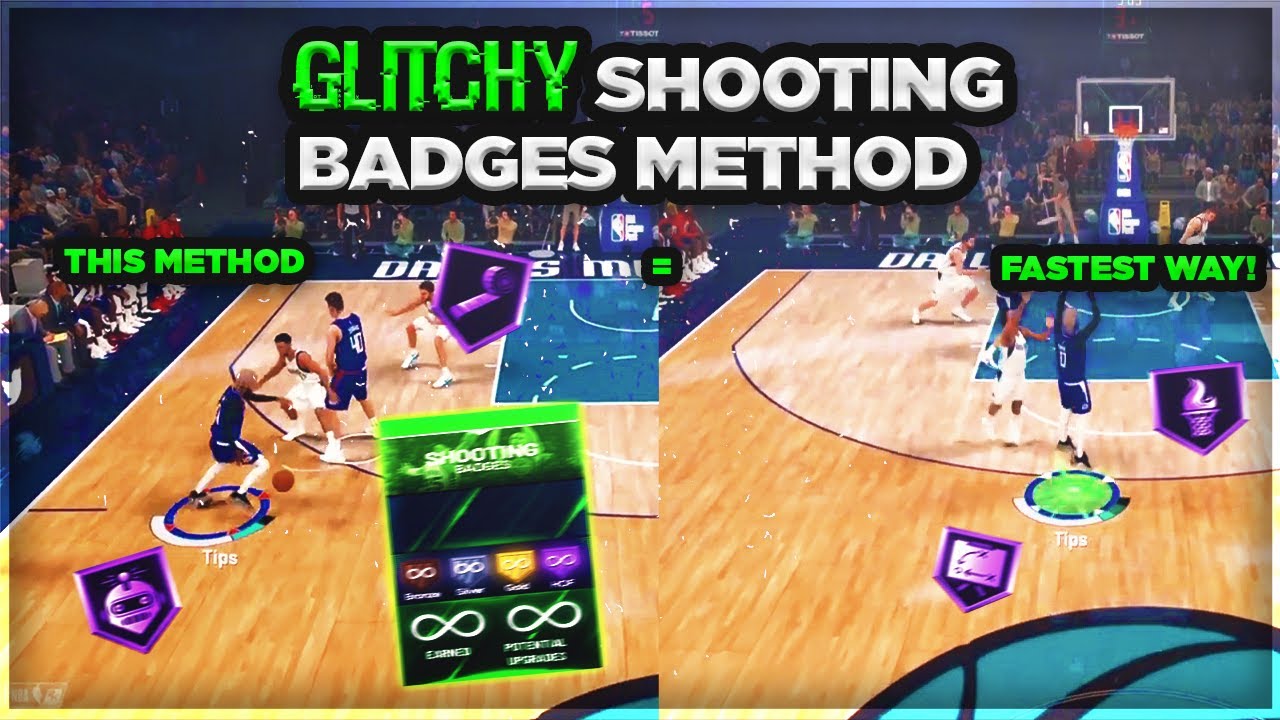The image captures two screenshots from a basketball video game, merged into one display.

**Left Side:**
- The background features an animated crowd.
- Across the top and down the left side halfway, there is a purple shield with a black border. Inside the shield is a purple robot head.
- To the right of the shield, a large green playing card bears the title "SHOOTING BADGES" in white at the top.
- Below the card's title, there are four badges: red, blue, yellow, and purple. The text beneath the badges is too small to discern.
- Beneath the badges, there are two infinity symbols in white, each accompanied by unreadable letters.
- The court action reveals two players in blue; one is dribbling to the right. Another player in white is guarding the dribbler, while a third blue player sets a pick.
- Another purple-bordered badge with a black interior and a roll of tape icon is visible.
- Bold green text in all capitals reads "THIS METHOD." Above it, extending across both images, bold green text reads "GLITCHY," followed by white text "SHOOTING BADGES METHOD," framed by a black border.

**Right Side:**
- The crowd remains visible at the top and left side of the screen.
- The basketball rim is now clearly seen near the right edge of the image.
- Two players, initially further away, have moved near the hoop. One defender in white, positioned to the left, raises his hand. The offensive player is centrally located, highlighted by a green circle with a blue border, preparing to shoot.
- Above the shooter, in bold green letters, "FASTEST WAY!" is prominently displayed.
- To the right of the player, there is a shield featuring a basketball engulfed in flames.

This caption offers a thorough description of the visual elements and context within the combined game screenshots.